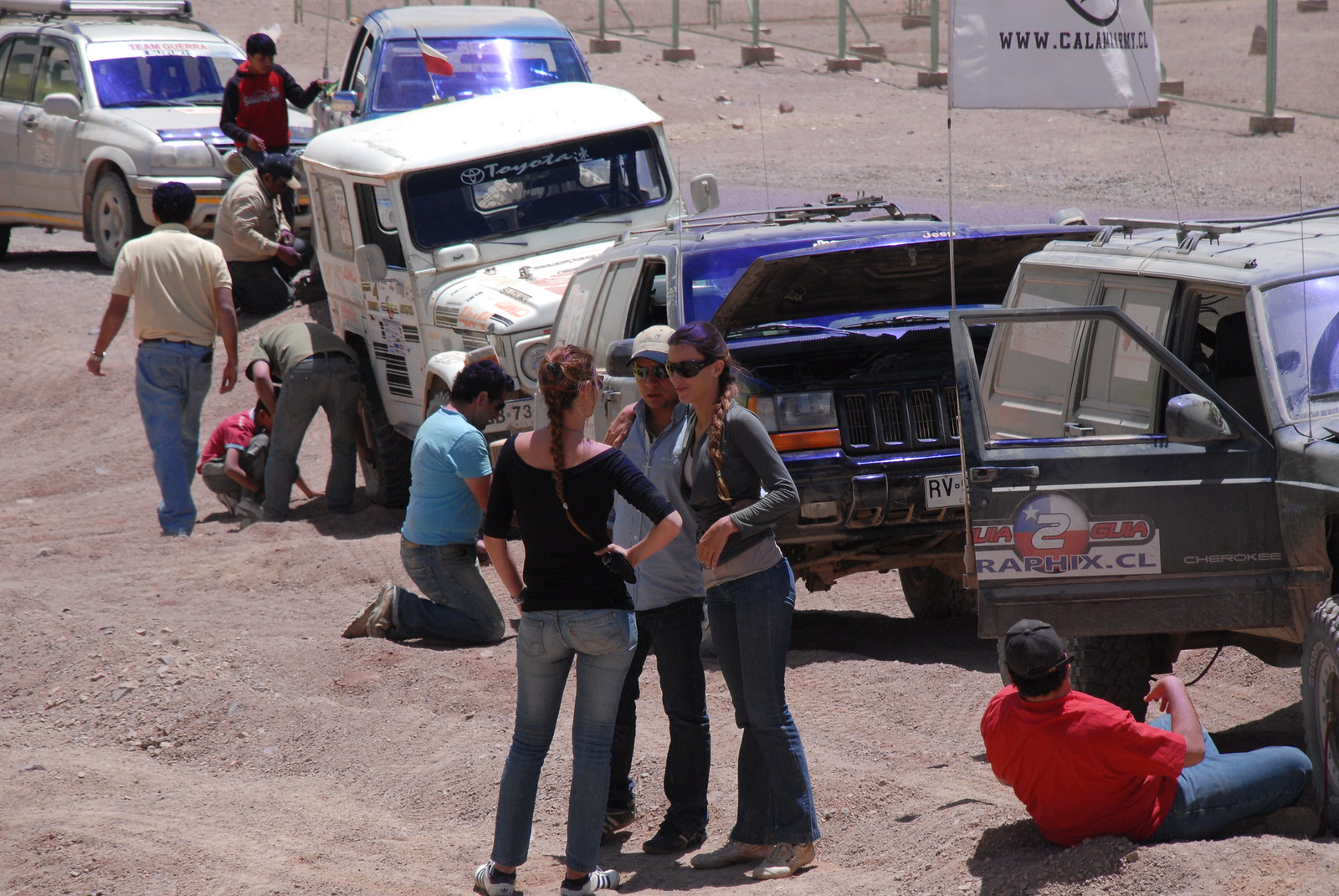This photograph captures a scene in a desert or dirt area where six vehicles, primarily SUVs and Jeeps, are lined up from front to back. The line is led by a dirty Jeep Cherokee, which bears the number two in a red, white, and blue circle with "RAPHIX.CL" beneath it. This lead vehicle has its passenger door open, revealing a man in a white T-shirt and blue jeans seated next to the door. Close by, three women are standing in conversation, with two of them having their arms around each other. Behind the first Jeep, another blue Jeep comes into view with a man in a blue shirt and denim jeans kneeling by the passenger door.

Further back, a white Toyota SUV can be identified by the name "Toyota" on its windshield. Three men are working on this vehicle; one is crouched down while the other two are standing. Following the Toyota, two more SUVs are lined up, including another white Jeep. People are seen near all these vehicles, either working on them or conversing. Additionally, a vehicle farther back displays a white and red flag. In the distance, a fence or gate is seen resting on cinder blocks, alongside some poles protruding from the ground. The scene is illuminated by sunlight, casting shadows on the ground.